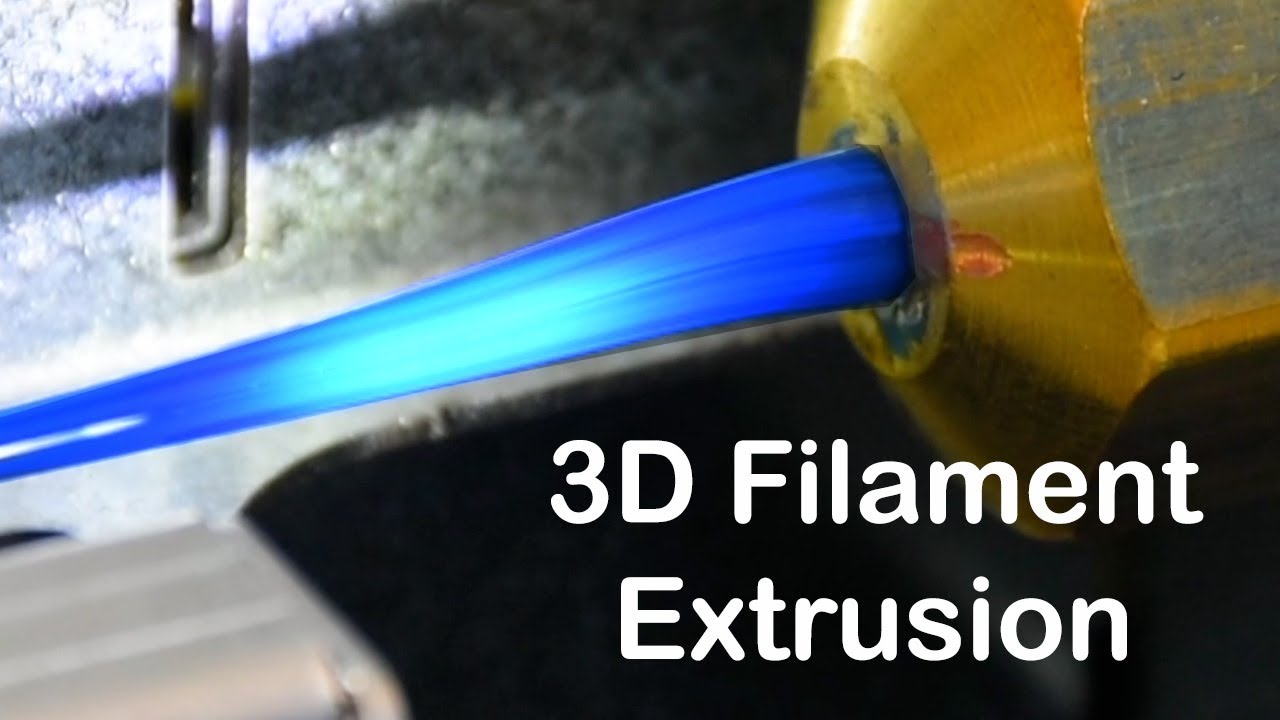The image depicts a close-up of a 3D filament extrusion process, emphasized by white text at the bottom right reading "3D Filament Extrusion." The focal point is a yellow and partially green mechanical device with a circular mouth, from which a blue, elastic-looking filament emanates. This filament extends and curves towards the upper left of the picture, suggesting it’s either being extruded or stretched. The device is situated in what appears to be a workshop, indicated by a gray, metallic background and possibly a wall. In the bottom right corner, the black section under the metallic device contrasts with the white text, making it stand out.